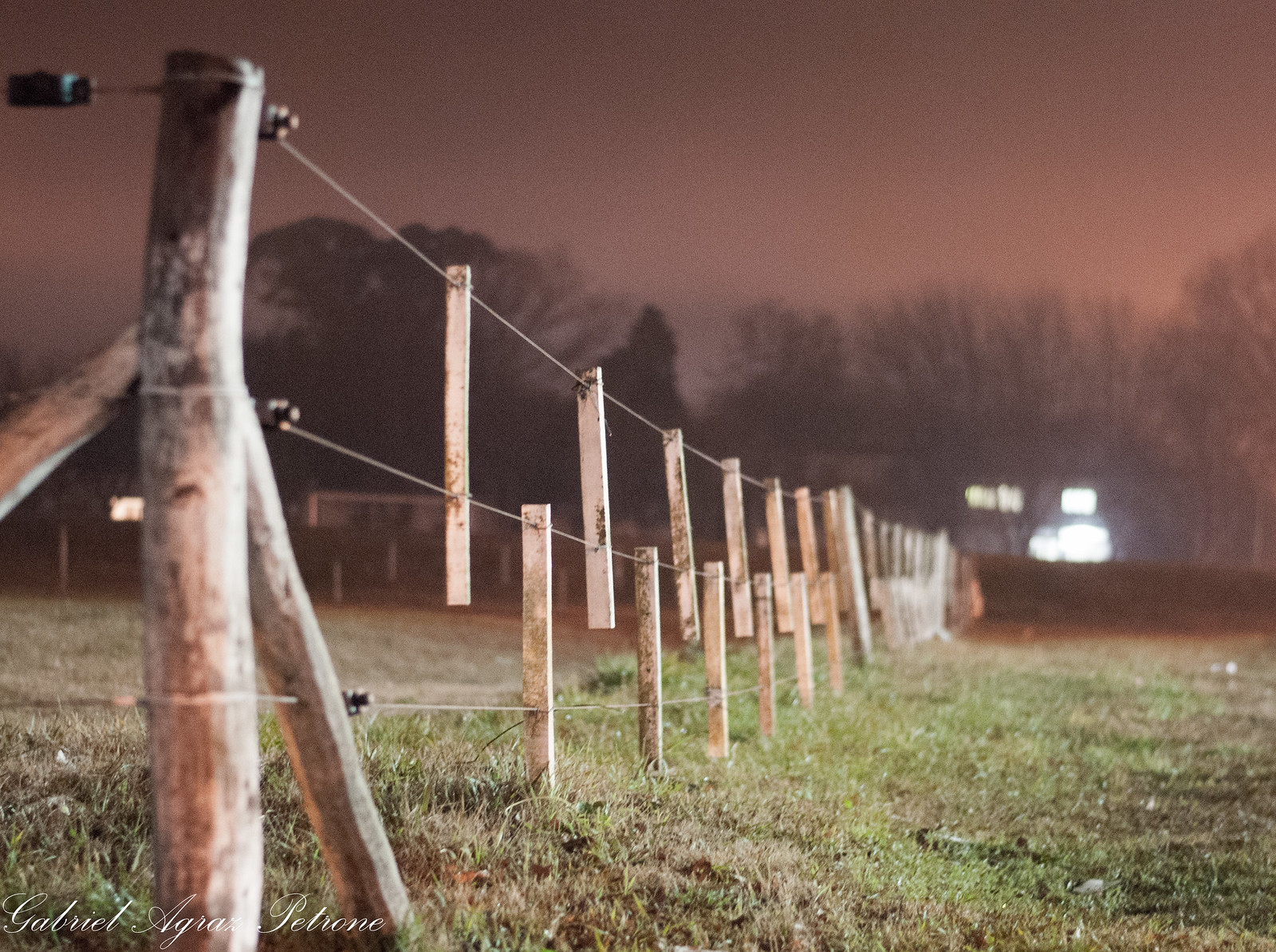The photograph captures an outdoor scene with a prominently featured farm fence stretching from the foreground to the background. The fence is constructed of alternating wooden posts, with three lines running across it horizontally—one near the top, one through the middle, and one near the bottom. The posts alternate in coverage: some extend from the ground to the middle wire and slightly beyond, while others span from the top wire down to midway between the middle and bottom wires. This pattern repeats six times before reaching a larger post that spans from top to bottom. The setting is a grassy farmland, set against a morning or nighttime backdrop with a sky darkened to an orange hue, suggesting either a sunrise or sunset. In the distant background, an illuminated house and garage can be seen near a dense line of trees. The fence posts are brown, and there seem to be black knobs attached to them. Additionally, there is text in the image, possibly bearing the name “Gabriel,” hinting at the photographer or author. The overall atmosphere is serene, with the green grass contrasting against the twilight sky and distant lights.